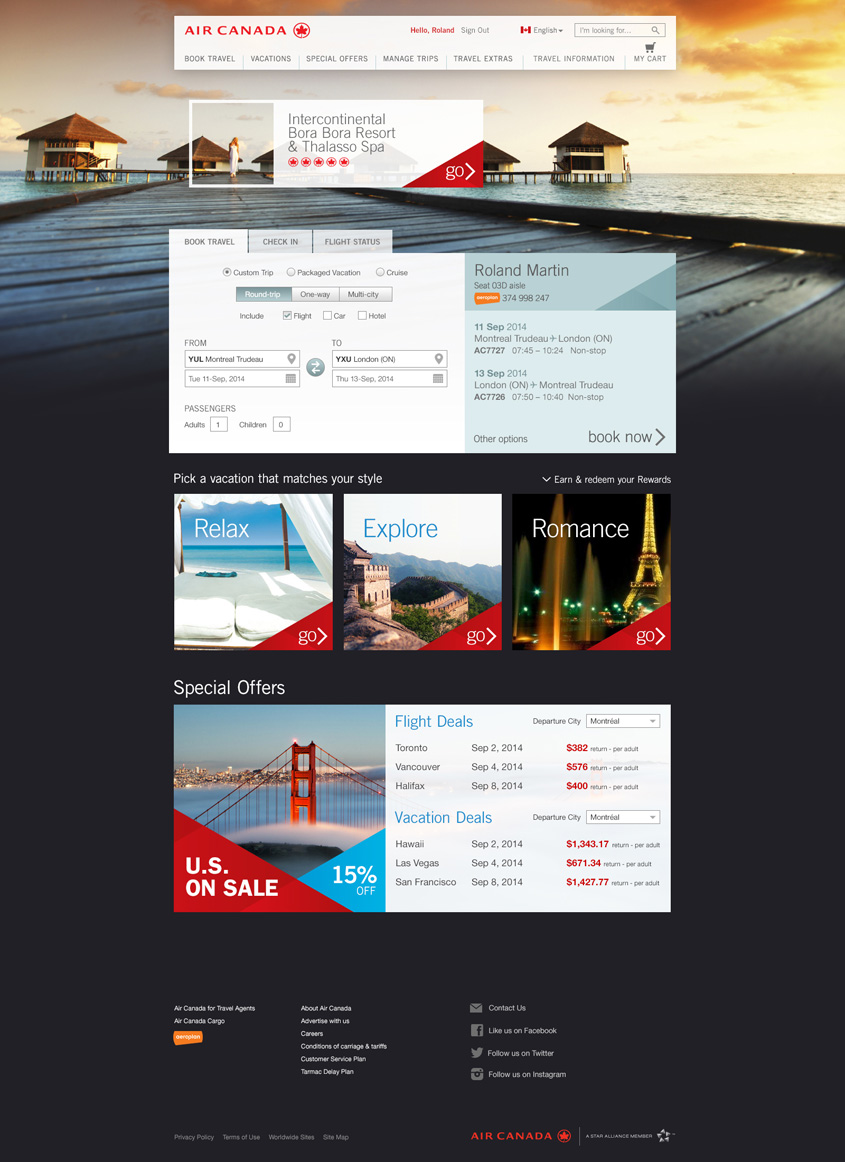This image captures the screenshot of a website featuring an evocative, immersive backdrop. The website's background displays a serene ocean scene with a dark gray dock extending out into the water, disappearing towards the upper left corner of the webpage. At the dock's end, quaint house-shaped structures with brown roofs and yellow siding add a touch of charm. The sky is illuminated with the vibrant golden hues of a sunset, creating a picturesque atmosphere.

Throughout the sky, a prominent white rectangle with bold, red "Air Canada" text stands out, accompanied by an icon of a five-pointed red star enclosed in a red circle. To the right of this logo, a search field invites user interaction, while various clickable options lie below: "Book Travel," "Vacations," "Special Offers," "Manage Trip," "Travel Extras," "Travel Information," alongside a car icon for transport-related needs.

Further down the page, a small banner attracts attention with the text "Intercontinental Bora Bora Resort and The Lasso Spa," accompanied by a five-star rating, suggesting luxurious accommodations. This banner seamlessly integrates into the website's immersive design, reinforcing the connection between the alluring image and Air Canada's travel services.